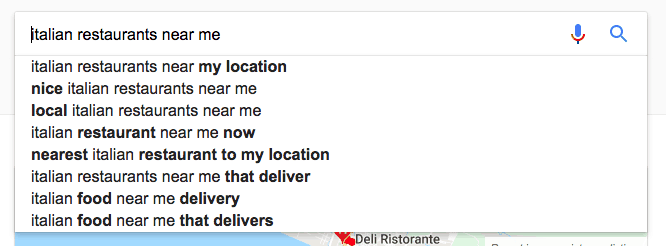The image captures a Google search result page with a query for "Italian restaurants near me." The familiar Google interface is evident through its distinct color scheme and search bar design. Within the search suggestions dropdown, additional related queries are listed, such as "Italian restaurants near my location," "Nice Italian restaurants near me," "Local Italian restaurants near me," "Italian restaurants near me now," "Nearest Italian restaurant to my location," "Italian restaurants near me that deliver," "Italian food near me that... delivery," and "Italian foods near me that delivers."

Behind the suggested searches, a partially visible map features a highlighted location labeled "Deli Ristorante." The search bar itself includes a blue microphone button with red accents, allowing users to conduct voice searches. Adjacent to it, the magnifying glass icon, also blue, serves as the search initiation button, which can be clicked after typing a query. The overall layout and elements of the page are characteristic of Google's intuitive design, aimed at providing a seamless search experience.